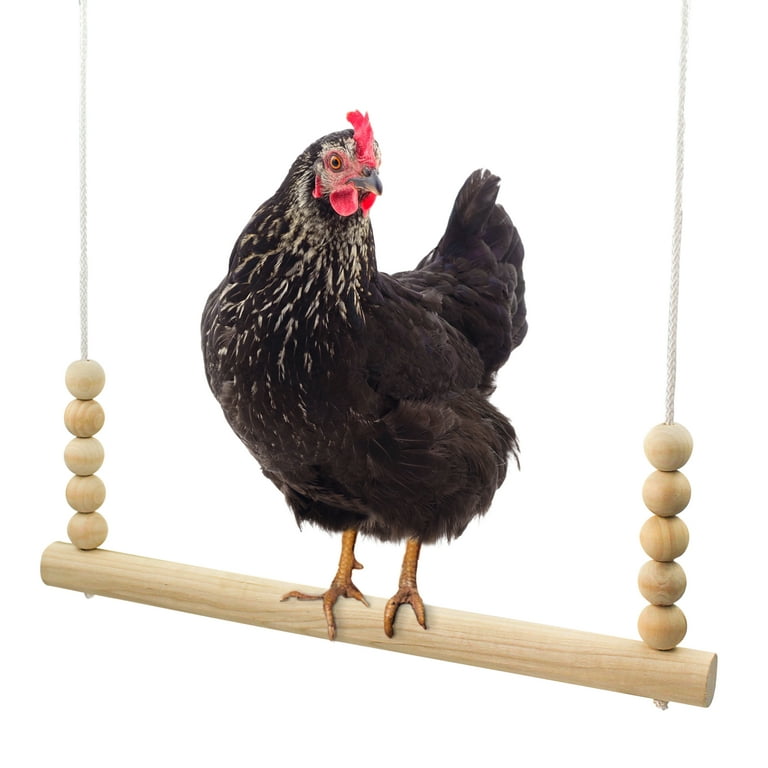In the image, we see a chicken with very dark brown feathers accented by white highlights stretching from its head down its neck, blending into its body. The chicken has a distinctive red comb on top of its head, complemented by matching red wattles hanging beneath its cheeks. Its eyes are striking—a golden orange with black pupils. The beak is mainly black, with some subtle beige coloration on the bottom. This chicken is looking towards the left side of the image. Its legs are yellowish-brown, securely perched on a light brown, unfinished wooden swing. The swing is made from a thick wooden dowel, supported by two white nylon ropes on each side. Each rope is adorned with five large, unpainted smooth wooden beads where they meet the dowel. The background of the image is a clean, solid white, emphasizing the chicken and its roost.